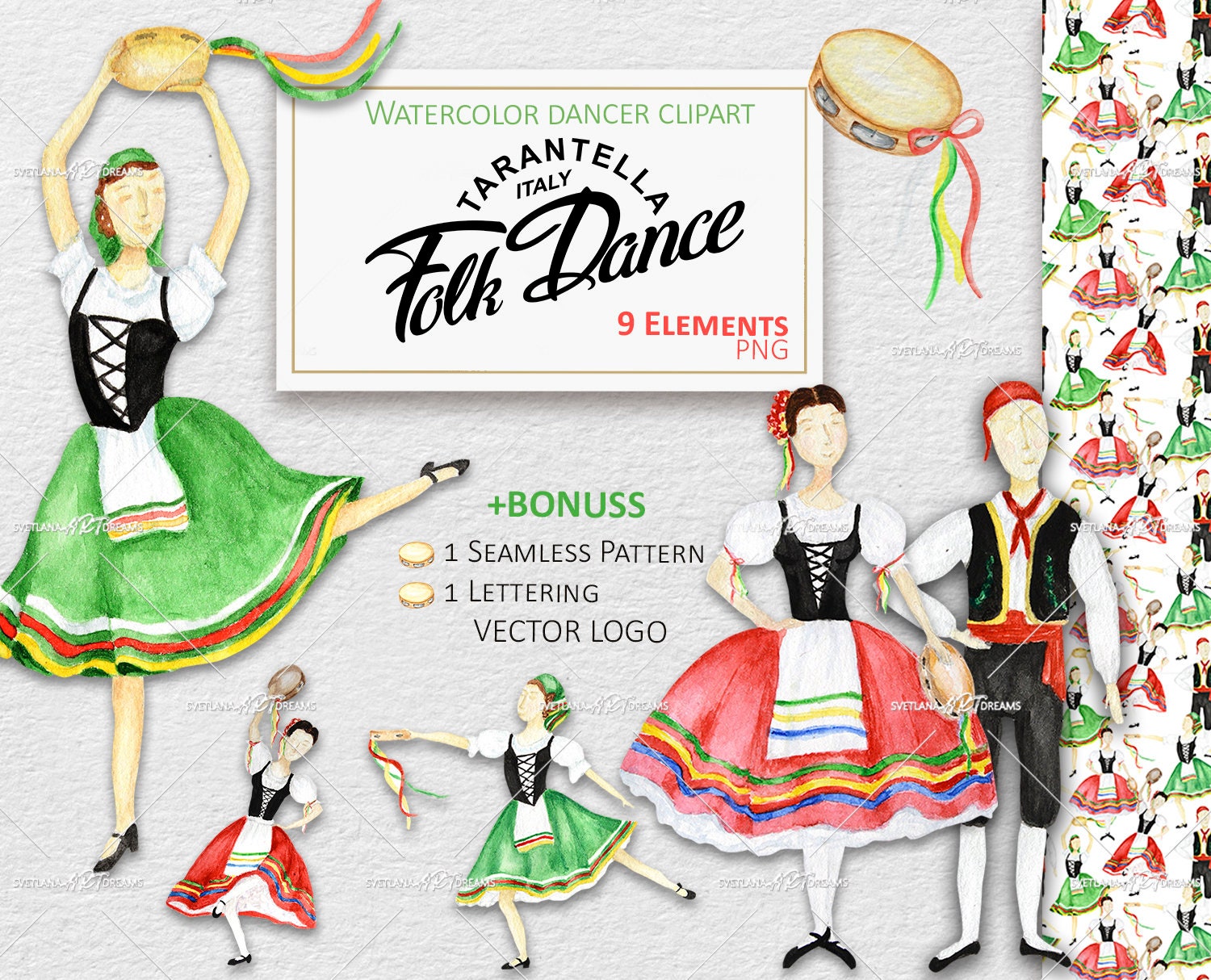This detailed advertisement showcases "Watercolor Dancer Clip Art" themed around the Italian Tarantella folk dance. Set against a gray background, the centerpiece is a banner with the title "Watercolor Dancer Clip Art - Tarantella Italy Folk Dance" emphasizing that the pack contains nine PNG elements. The central text also highlights a bonus that includes "One seamless pattern, one lettering vector logo," with the word "bonus" conspicuously spelled with an extra 'S' (bonusS).

To the left of the banner, there's a prominent figure of a female dancer dressed in traditional Italian attire—a green skirt paired with a white bodiced shirt and a black front bodice—holding a tambourine above her head. Near her, a tambourine adorned with red, yellow, and green ribbons adds a splash of color. Beneath the banner, additional illustrations include two smaller images of dancers. On the bottom right, a male and female pair echoes the traditional garb, enhancing the cultural theme.

Embedded throughout the design, watermark text "Svetlana Dreams" subtly brands the product while various watercolor illustrations of Italian folk dancers in vibrant green and red skirts with bolero-style outfits and tambourines create a rich, repeating pattern in the background. This visual combination recreates the lively spirit of the Tarantella dance, making it a captivating choice for users seeking festive and cultural clip art.